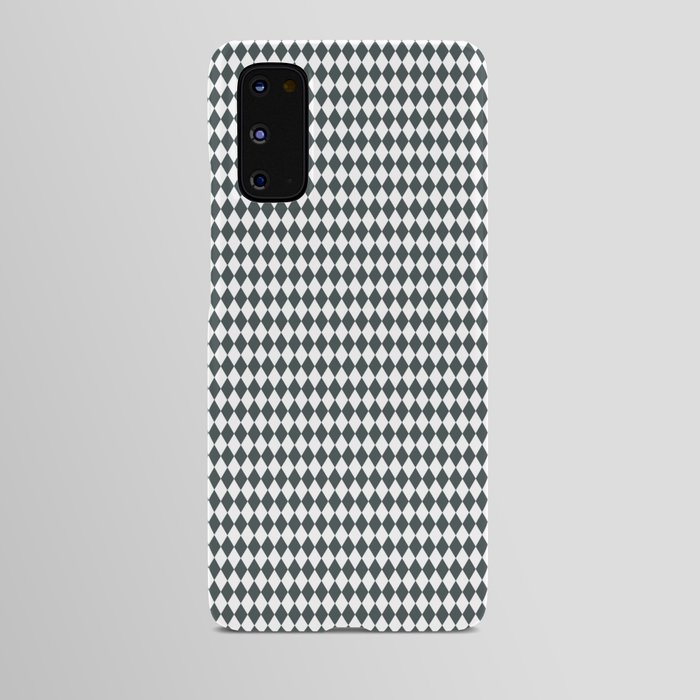The image displays a detailed mock-up of an iPhone case set against a light gray background that gradually darkens towards the left side and lightens at the bottom right corner. The iPhone case features a sophisticated pattern of interconnected, small diamond shapes arranged in rows of gray and white, forming a visually appealing checkered design that extends from top to bottom and left to right across the case. The iPhone, which is relatively thin, has a vertically-aligned tri-camera system at the top left, identifiable by three distinct blue lenses each encircled by varying shades of gray rings. The case covers the entire back of the phone, emphasizing the elegant gray and white diamond motif without any additional text or markings.